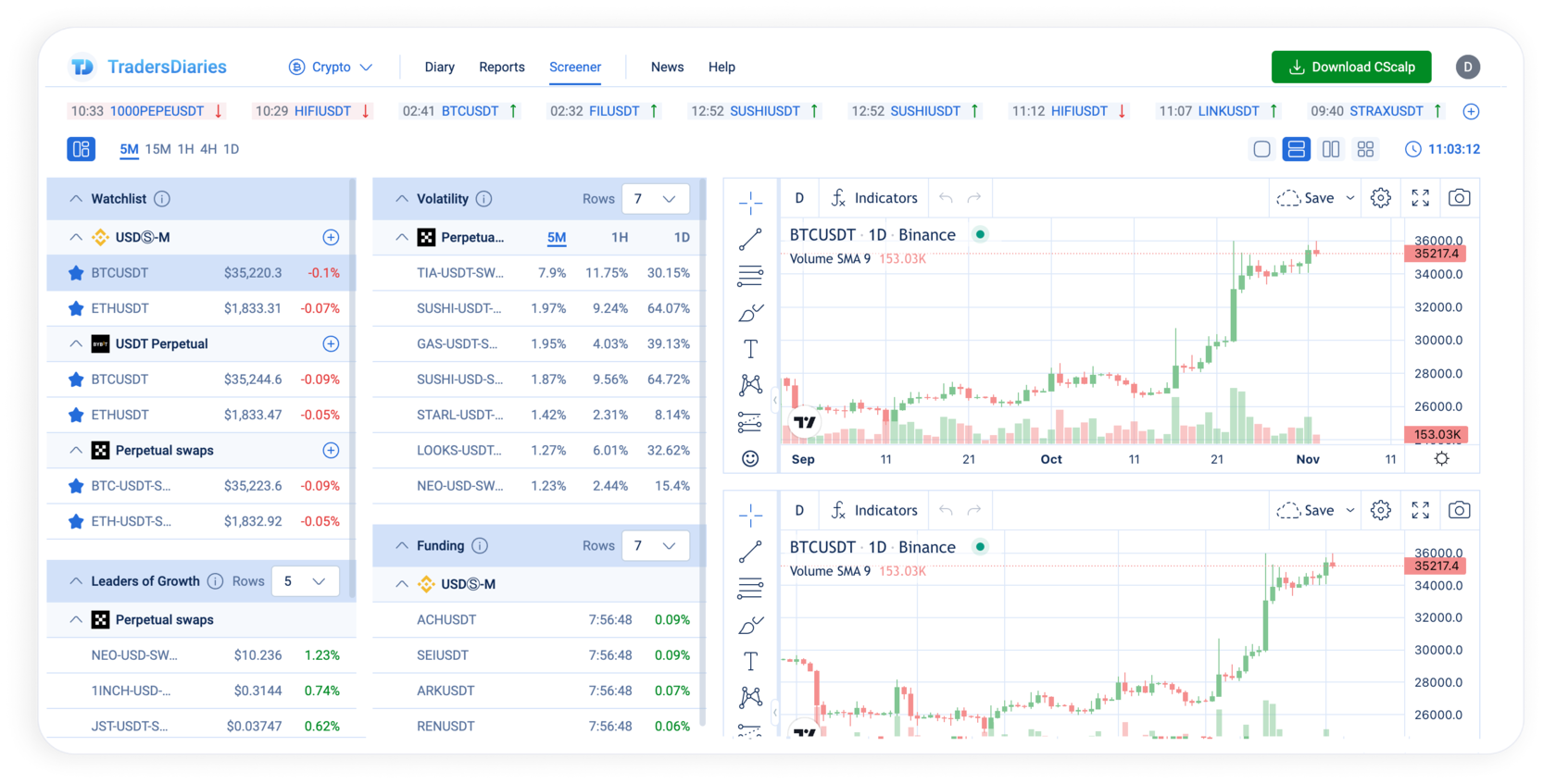The trading chart displayed is part of a cryptocurrency-focused platform named "Trader's Diaries," prominently indicated in the upper left-hand corner. It features a dropdown menu allowing for selection among various categories with "Crypto" currently chosen. The interface offers several functions including Diaries, Reports, Screener, News, Help, Download, See, and Scalp. 

The central focus is on the Bitcoin versus U.S. Dollar trading data, depicted with green arrows for price increases and red arrows for declines. Directly below this, there's a watchlist comprising approximately ten selected items. Adjacent to the watchlist are sections titled "Leaders" and "Growth," indicating significant market movers.

To the right of this setup lies another column dedicated to "Volatility," highlighting the most volatile assets and details about funding rates. The chart section to the far right presents various chart indicators and analysis tools specific to Bitcoin and U.S. Dollars. Two primary charts are displayed, stacked vertically and appearing to show identical data visualizations. These charts use vertical green and red bars to indicate the trading range for each day, confirming them as daily charts.

The overall color scheme of the platform is predominantly blue and white, with the charts themselves utilizing green and red to represent different market movements. The interface is data-rich, making it a bit overwhelming to digest all at once.